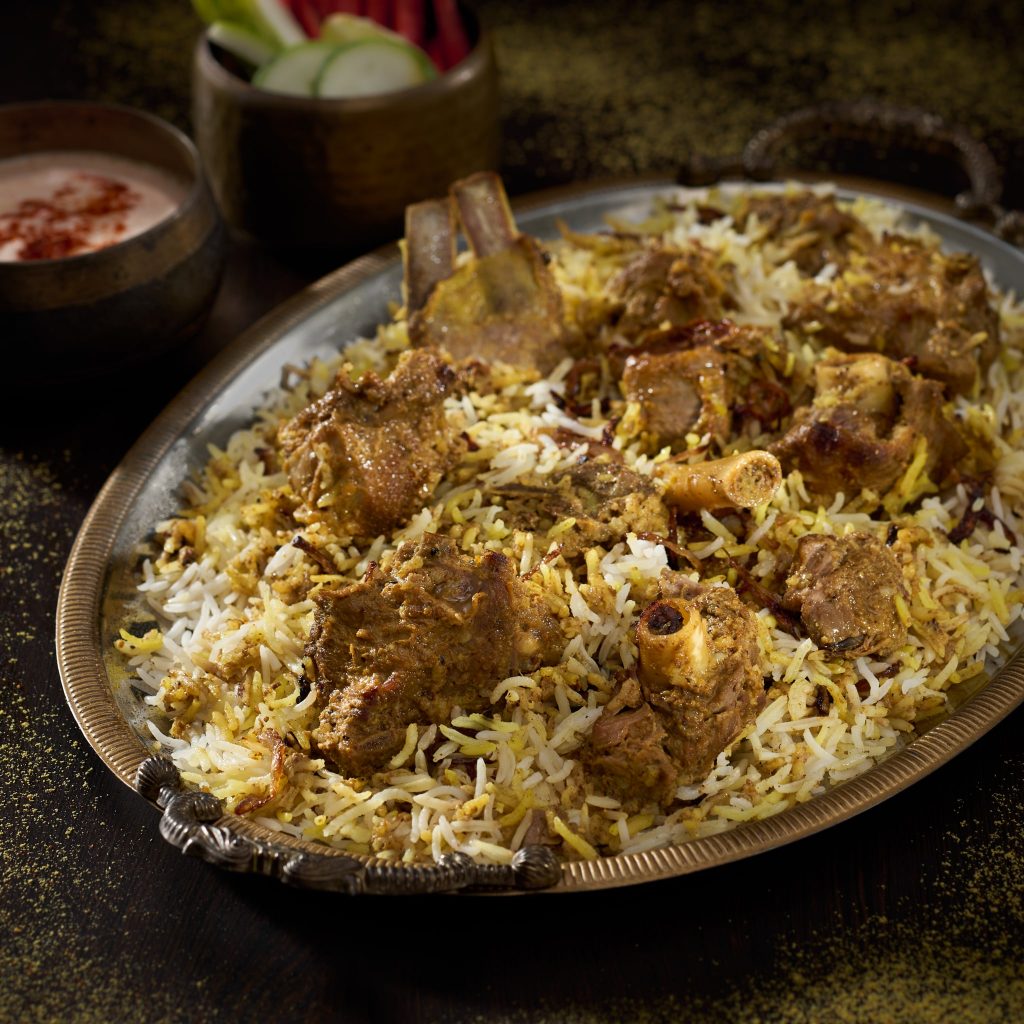The image depicts a large, gold-colored serving dish filled with a bed of long-grain rice, likely biryani, showcasing shades of yellow and white. On top of the rice, there are succulent short ribs with visible bones protruding, each with a small amount of roasted brown meat attached. The dish is the focal point, while in the blurred background to the top left, there are additional bowls, one containing vegetables and another with a creamy yogurt or chutney. The setting of the photograph suggests an ambiguous time of day and location, possibly taken on a dark blanket. The overall color palette includes white, light yellow, brown, dark brown, green, red, maroon, and gray.